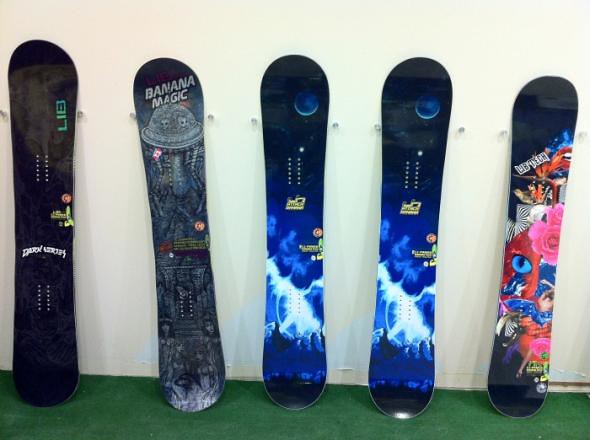The image depicts five skateboards leaning against a white wall, supported by pegs sticking out to hold them upright. The skateboards are all lined up on green carpeting. From right to left, the first board is the most colorful, featuring a black background with a pink flower, an orange creature with a blue eye, and various abstract patterns in red, orange, and blue, giving it a vibrant and tech-inspired appearance. The second and third boards are identical, featuring a design that resembles a dark blue sky with white clouds and mountains, transitioning to black at the top with a blue moon; these boards have rounded edges and a striking visual of a blue and white scene. The fourth board has "Banana Magic" written in pale white on a dark gray background, and features what appears to be a gray spaceship or a dome with eyes. The board on the far left is almost entirely black with lime green letters that spell "L18" or something similar, accompanied by other indistinct white lettering and round dots forming lines. The environment, due to the white wall and pegs, suggests an indoor setting, possibly even a ship's interior.